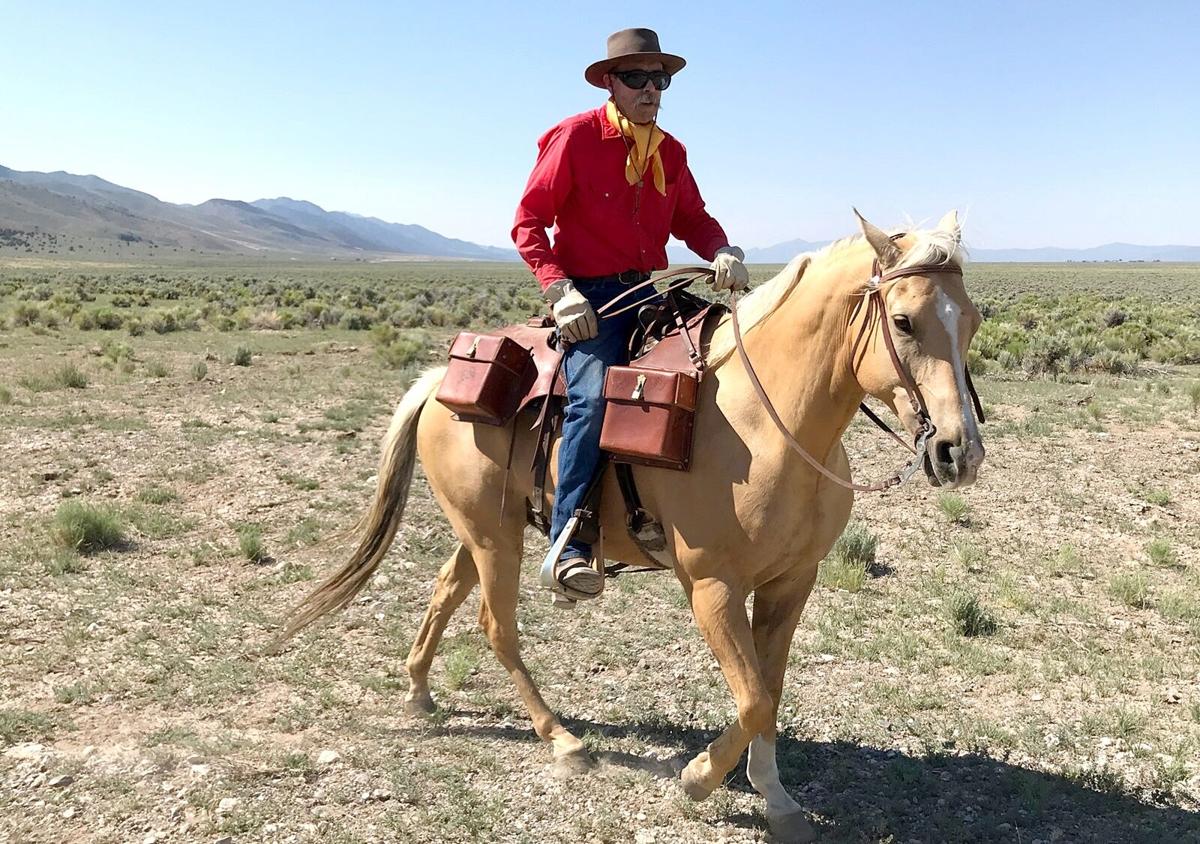The image depicts a man riding a light brown horse with a distinctive white stripe running from its nose up to its forehead. The horse has small ears and a white mark on one of its hooves. The man is dressed in a bright red shirt with a bright yellow handkerchief tied in a bow at his neck, blue jeans, and white gloves, while his face is partially obscured by sunglasses and a handlebar mustache. He wears a small-brim cowboy hat and boots that rest in the stirrups of the saddle. The saddle is red and features leather pouches on either side. The scene is set in an open, desert-like landscape with patches of green shrubs scattered across the ground. In the background, there is a distant mountain range that appears grayish due to atmospheric effects, all under a clear blue sky.